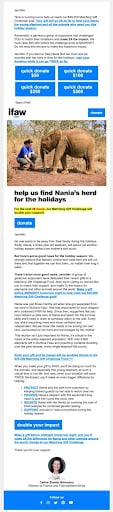The image appears to be a screenshot taken from a computer screen. At the top of the screenshot, there are three paragraphs of text, followed by four blue buttons that look like they might be donation buttons. Unfortunately, the text becomes increasingly blurred as you zoom in, making it difficult to read. Below these buttons, there is a photograph featuring an elephant standing outdoors on brown dirt, framed by trees and a clear sky in the background. The elephant is looking to the left, where a person dressed in a blue t-shirt and gray pants is kneeling in front of it. 

Accompanying the photo is a caption reading "Help us find Nana's herd for the holidays," with another blue button labeled "Donate" situated underneath. Following this, there are six to seven paragraphs of text that provide additional context or information. At the end of this block of text, there is another blue "Donate" button. Finally, at the bottom of the image, there appears to be a picture of a person, likely the author of the article.